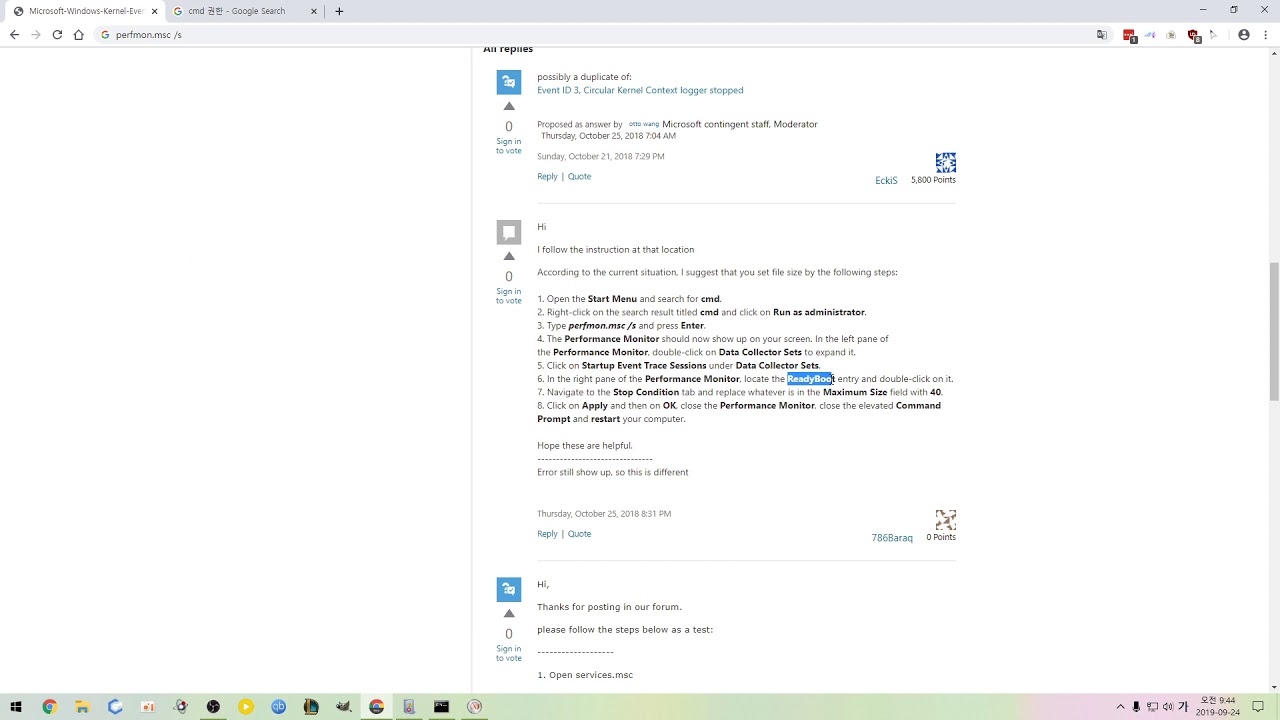This horizontal image, likely a screenshot taken from a computer screen, depicts a webpage with various elements of a browser interface. At the top, there's a white bar indicating the web page's title in Microsoft Edge or another Microsoft-related content. Below this title bar is a long, thin, gray rectangular bar displaying the browser's window controls, including minimize, maximize, and close buttons on the top right.

On the top left, the browser features navigation elements such as back and forward arrows, a home icon, the web address bar, and additional icons situated on the upper right. The majority of the screen is white, suggesting an uncluttered background typical of a web document or forum page.

The right and middle sections of the image provide detailed content of the web page being viewed. This section appears to show a forum or discussion thread. The forum entries suggest a dialogue involving troubleshooting or technical support. Phrases like "possibly a duplicate of," "hi, I followed the instruction," and "according to the situation" indicate an ongoing conversation, with participants offering detailed steps to resolve an issue. One participant's response includes a list of steps aimed at addressing a file size problem, closing with a polite "hope it helps," while another person acknowledges the inquiry and suggests a test with further instructions.

Below the main content area, the bottom edge of the image showcases part of the user's computer taskbar, indicating the various applications and options available for them to interact with.